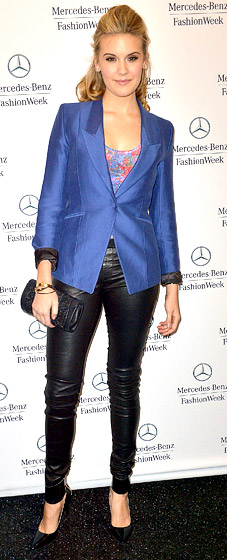The photo captures Maggie Grace standing elegantly before a white backdrop adorned with the Mercedes-Benz Fashion Week logo repeated in a pattern. She is poised on a black marble-like floor with white accents, clad in striking high-heeled black leather shoes. Maggie is wearing tight black leather ankle pants that accentuate her slender legs. Her attire is topped with a blue blazer, underneath which is a colorful shirt featuring a mix of blue, orange, and pink hues in a flowery pattern. Her dirty blonde hair is styled up and pulled back neatly behind her neck. In her right hand, she holds a black clutch purse, complemented by a gold and black bracelet on her wrist. Maggie’s dark eyes and poised stance add to her refined appearance at this fashion event.